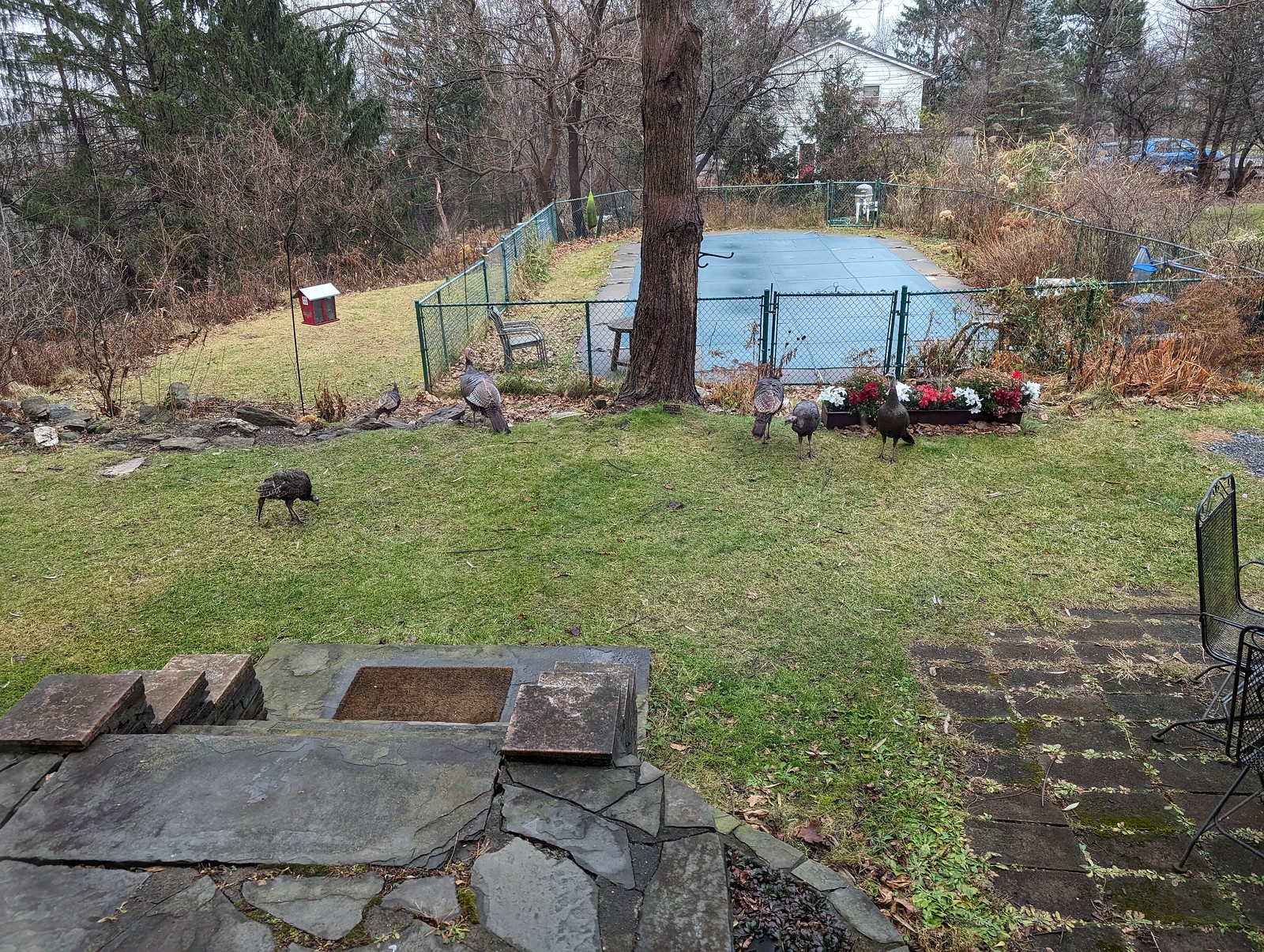The image depicts a spacious backyard, likely in a forested neighborhood, taken from the stone patio of a home. At the forefront, there's a small garden with neatly arranged plots bordered by grass, and some steps leading down. Scattered across the scene are several dark-feathered birds, possibly turkeys, though they could be peacocks due to the distance making identification difficult. There is a tall tree with a thick trunk prominently in the middle of the yard, with white, red, and pink flowers planted around its base. 

A blue-tarp-covered pool, surrounded by cement and enclosed with a green fence, is seen towards the center. Next to the pool is a chair and a table. A red birdhouse is perched visibly among the foliage. In the distance, beyond the green canopy of trees, a neighboring white-sided house is partially visible. The entirety of the scene evokes a serene, rustic atmosphere, typical of a countryside home.